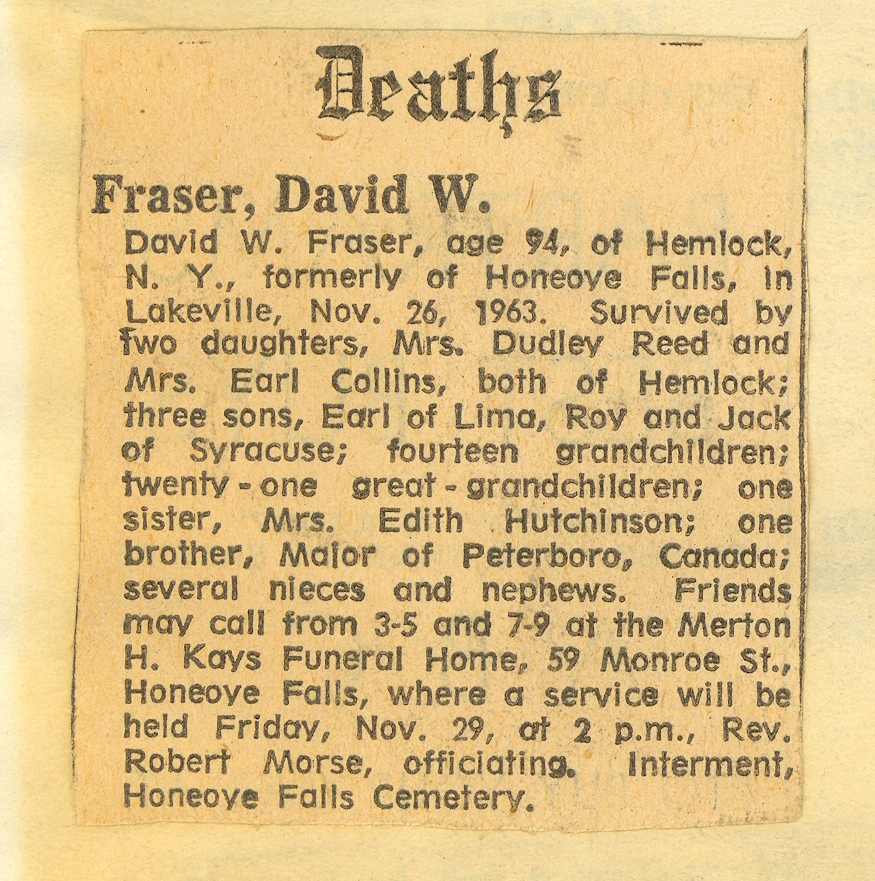The image depicts an old newspaper clipping from the obituary section, meticulously pasted on a mounting board. The aged paper has a beige hue, and the headline "Deaths" is displayed in an old-style font. The notice concerns David W. Frazier, age 94, of Hemlock, New York, formerly of Hunro Falls in Lakeville, New York, who passed away on November 26, 1963. He is survived by two daughters, Mrs. Dudley Reed and Mrs. Earl Collins, both of Hemlock, and three sons, Earl of Lima, and Roy and Jack of Syracuse. Additionally, he is remembered by his 14 grandchildren, 21 great-grandchildren, one sister, Mrs. Edith Hutchinson, and one brother, Maylor of Peterborough, Canada, along with several nieces and nephews. Friends may call from 3 to 5 p.m. and 7 to 9 p.m. at the Merton H. Kays Funeral Home, located at 59 Monroe Street, Hunro Falls. The funeral service is scheduled for Friday, November 29th at 2 p.m. at the Falls Cemetery, officiated by Reverend Robert Morse.